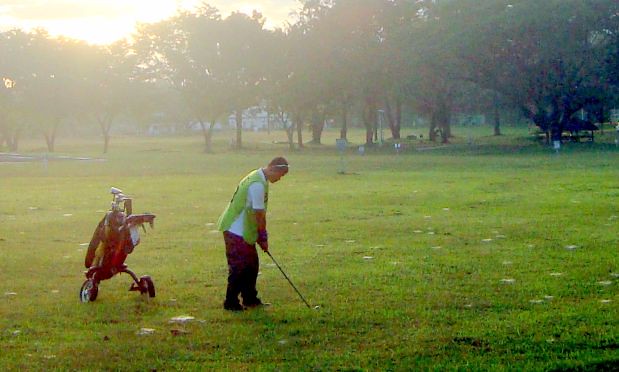In this rectangular outdoor photograph, taken either at dawn or dusk, the sky is tinged with a golden light as the sun hovers halfway above the horizon. The scene unfolds on a well-trimmed golf course, characterized by its lush, green grass speckled with light-colored patches which might be flowers or patches of sunlit grass. In the background, a sparse line of trees with dark trunks and green leaves borders the grassy area.

Central to the image stands a gentleman, poised in mid-action, holding a golf club as if preparing to hit the ball. He is dressed in a white t-shirt layered with a green vest and wearing dark pants. Beside him rests a bag of golf clubs mounted on a handy two-wheeled cart, ready to be easily pulled along. Despite the serene and somewhat picturesque setting, the grass shows marks from numerous past hits, suggesting an unevenly maintained course.

The area around him is mostly empty, save for a few distant figures and a mysterious basket by a tree, hinting at other unseen activities. In the extreme background, vague structures or possibly a clubhouse can be discerned, blending subtly into the mellow light of this tranquil golfing scene. The overall atmosphere conveys a moment frozen in time, capturing the quiet anticipation and solitary focus of the golfer amidst the peaceful surroundings.